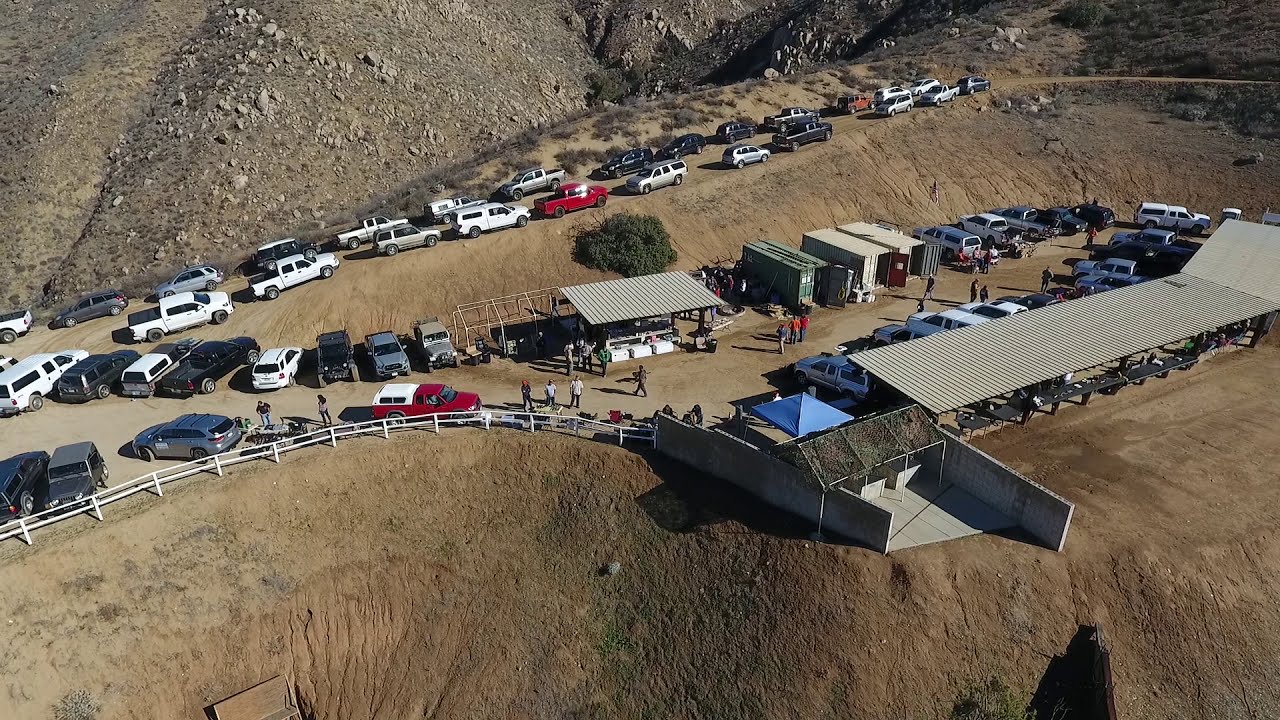The image shows an aerial view of a dirt-paved parking lot situated on the side of a rocky, sandy hillside or cliff, characterized by its light brown terrain and multiple layers. Prominently visible in the foreground is a steep drop-off or pit, enclosed by a white barrier fence that serves to prevent dangerous falls. Rows of cars are densely parked on both sides of the dirt driveway and along a nearly parallel dirt road higher up the hillside. Among these parked vehicles, which come in various colors like white, red, silver, and blue, there are also covered awnings or railing structures providing some form of sun protection. Nearby, storage containers with their doors open suggest that the area may function as a worksite, although this is not certain. This combined scenery, framed by a precarious mountain setting and the protective white fencing, underscores the area's ruggedness and the necessity for safety precautions.